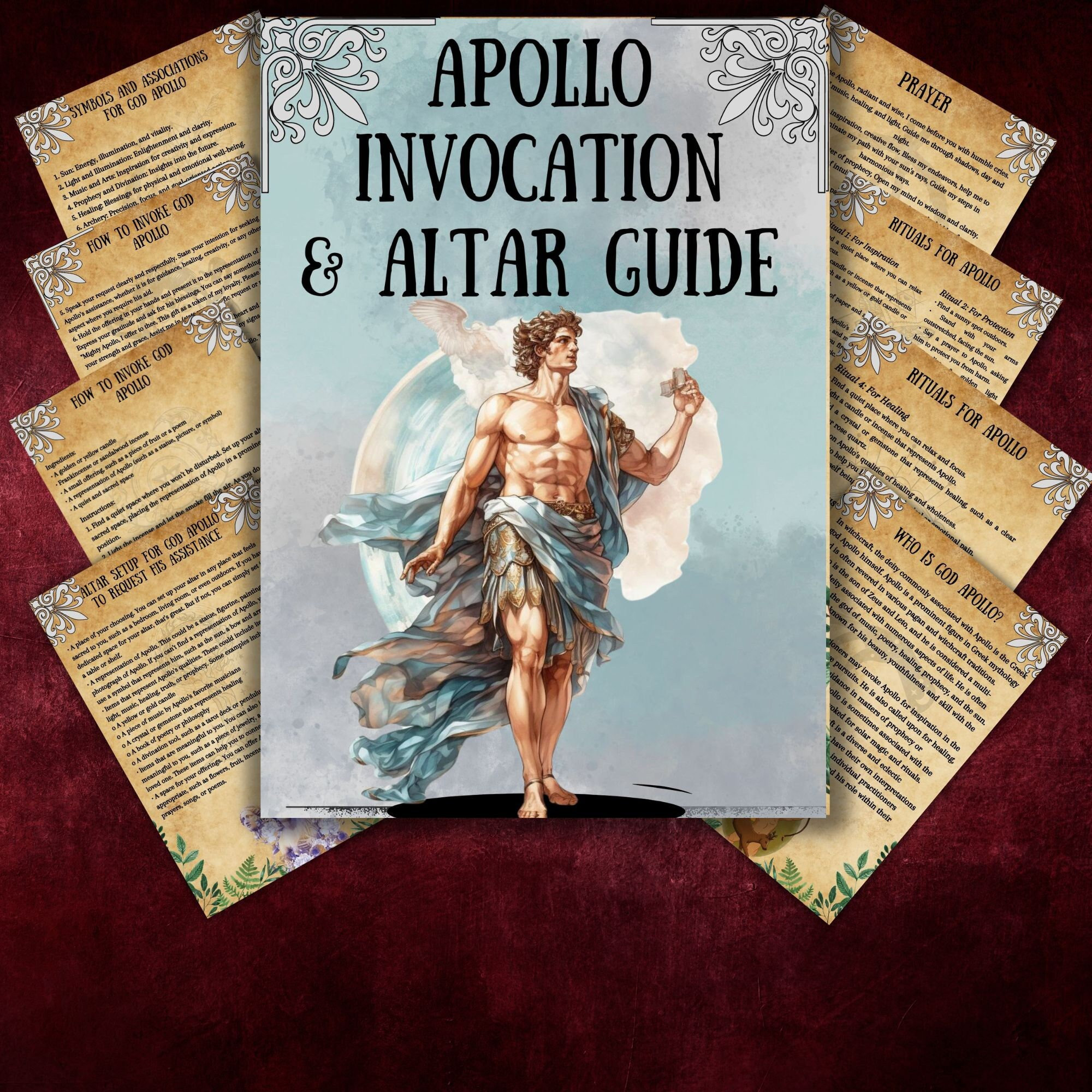The large square picture features a velvety reddish-brown background. At the center top, there is a vertical rectangular image with the title "Apollo Invocation and Altar Guide" written in all caps, black letters. Just below the title, a muscular, tan-skinned depiction of Apollo dominates the image. He has curly brown hair and is bare-chested, draped with wavy, blue and brown cloth over his shoulders and waist. A cloud appears to be behind him, suggesting a sky background.

Flanking Apollo and the main guide are eight diagonal sheets of paper or cards, four on each side. On the left side, arranged from top to bottom, the titles read:
1. Symbols and Associations for God Apollo
2. How to Invoke God Apollo
3. How to Invoke God Apollo Again
4. Altar Setup for God Apollo to Request His Assistance

On the right side, the titles are:
1. Prayer
2. Rituals for Apollo
3. Rituals for Apollo Again
4. Who is God Apollo?

This detailed and ornate arrangement highlights various aspects of invoking and venerating the Greek god Apollo.